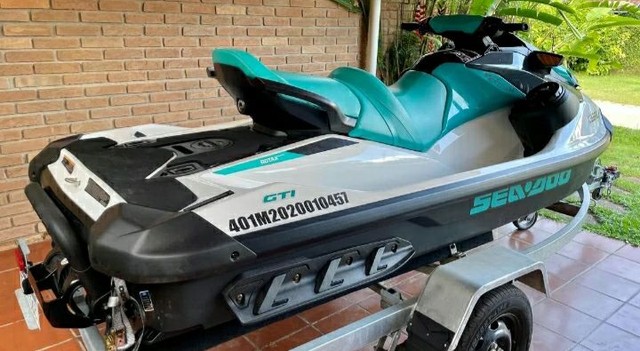The image showcases a Sea-Doo jet ski positioned centrally on a gray, aluminum pull-behind trailer in a carport beside a brick house. The jet ski is viewed from the side, highlighting its teal, black, and white color scheme. The teal seat, designed for two riders, complements the matching center green handle grips. The jet ski's body also features a black base and white accents, with "GTI401M20200010457" and "Sea-Doo" emblazoned in teal letters on the side. The setting includes a ceramic-tiled floor in a brown or orange hue inside the carport, with green grass and shrubbery visible in the front and a walkway leading to the house. A silver hitch extends to the right side of the trailer, which sits in proximity to a downspout on the brick wall.